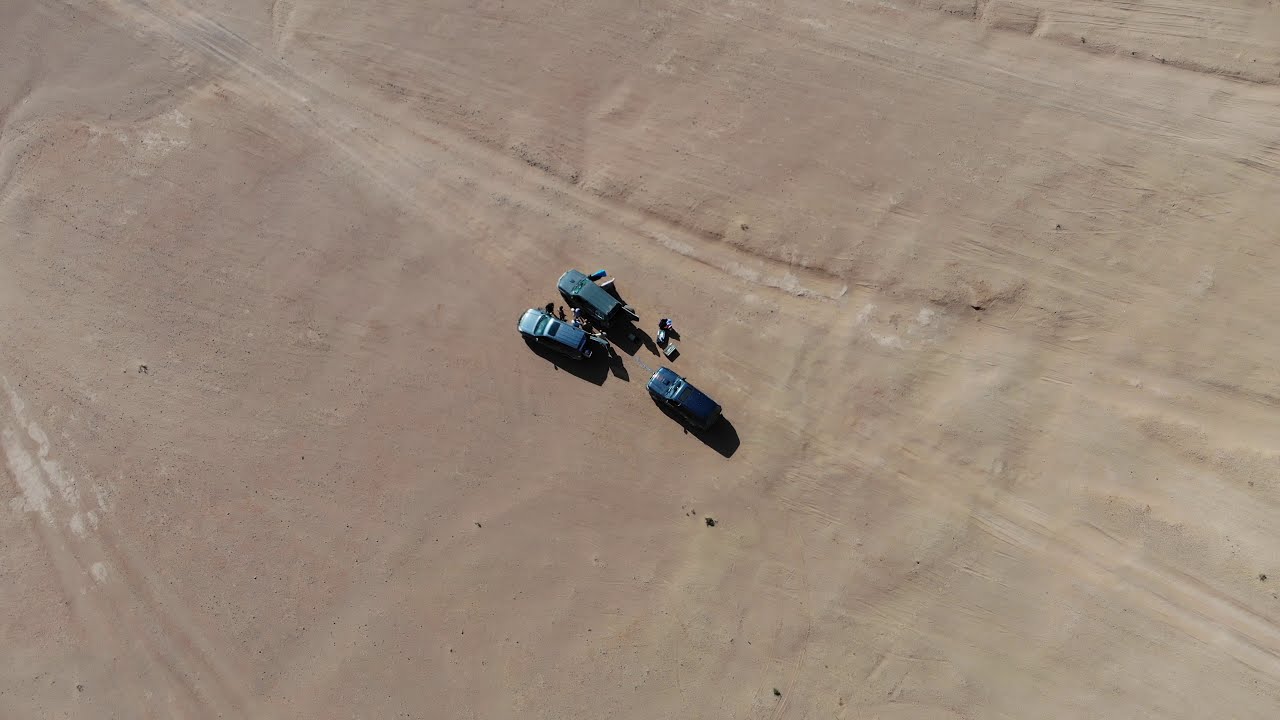This captivating aerial image, taken during the daytime, features a desert scene with hard-packed, darker tan sand dotted with small rocks and deeply carved tire tracks stretching diagonally from the lower right to the upper left of the frame. In the midst of this desolate landscape, we see three vehicles and a navy blue van positioned in a staggered formation, creating a dynamic focal point. The vehicles include a dark forest green truck in the foreground and a blue truck to its left, while the navy blue van lingers towards the back. Between the vehicles, camping equipment or various bags are strewn about on the ground, hinting at a recent or current outdoor adventure. Closer inspection reveals what might be tiny figures or toys, suggesting the entire scene could be a meticulously arranged set rather than a real-life scenario, playing a trick on the eye.